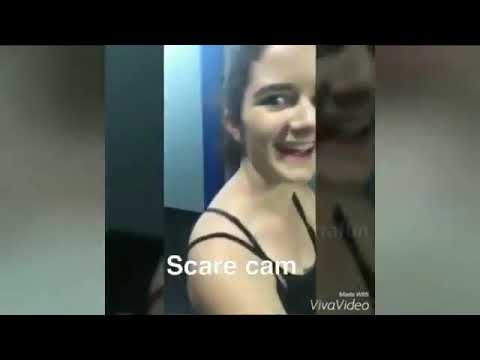The image is a screen capture of a video featuring a young Caucasian woman with dark hair and dark eyes, smiling directly at the camera. She is wearing a black tank top with thin spaghetti straps. The image appears to be set indoors, likely in the middle of the day. In the background, there is a visible floor and wall, but no other objects stand out. The photograph has black horizontal borders at the top and bottom, reminiscent of widescreen video bars. The main image is centrally positioned, with a zoomed-in version of the woman’s face slightly larger and darker behind it. The bottom of the image displays the text "scare cam" in white letters, just above "made with VivaVideo" on the bottom right. The overall color palette includes tan, green, black, blue, and white.